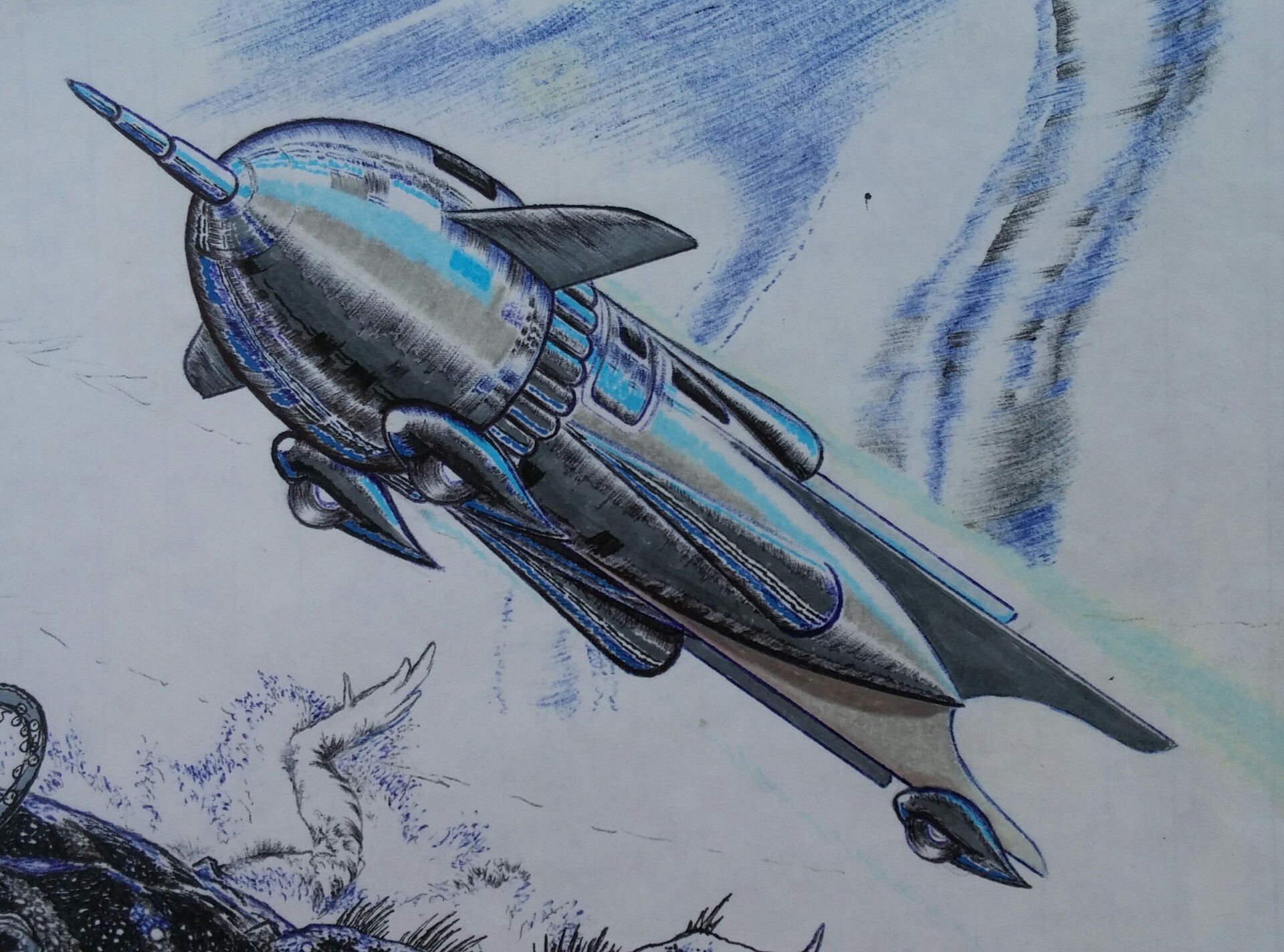This image features an artist's rendition of a silvery rocket ship with blue and turquoise streaks that match the whitish background with similar blue elements. The rocket is depicted mid-takeoff, oriented sideways in the air, with a distinct, pointed tip resembling a unicorn's horn at one end and traditional rocket fins at the other. The backdrop showcases a sky filled with cloud-like formations, with an impression of a tornado-like swirl. Below the airborne rocket, there appears to be part of the ground and an animal leg, which is reminiscent of a Dr. Seuss character with a small foot, hair, and three toes, seemingly reacting to the rocket's ascent. The scene intricately blends imaginative and whimsical elements, making for a visually intriguing composition.